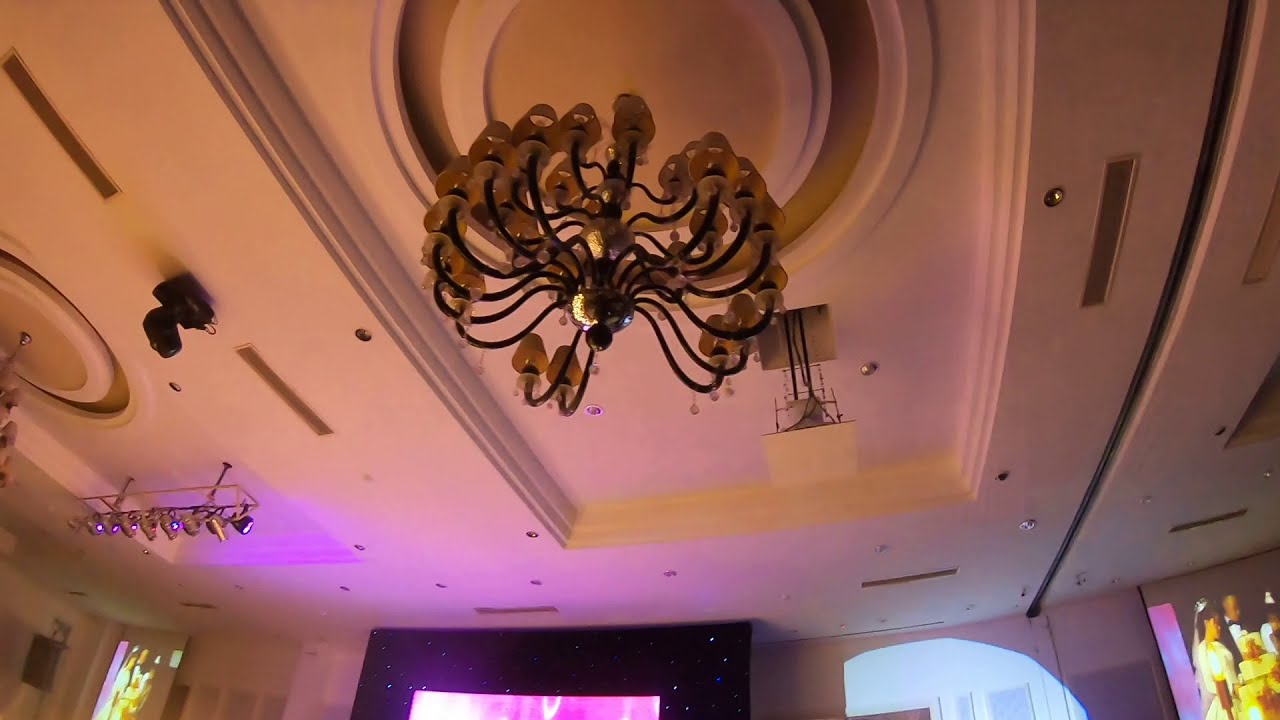This detailed interior photograph captures the ceiling of a ballroom or function room, viewed from below. The ceiling, primarily white, features an intricate design with a raised embossed circular molding. Within this circle, a grand chandelier, with more than 10 delicate light fixtures, hangs elegantly. Each light fixture is adorned with its own beige-colored lampshade, and the main metal structure is a dark black or brown. Scattered across the ceiling are recessed lights, adding to the elaborate decor.

The room is dimly lit, with a hazy purplish hue projected onto parts of the ceiling, contributing to an ambient atmosphere. Towards the right side, a large track is visible, suggesting a retractable divider feature. The ceiling's design also includes a rectangular recessed area encompassing the central circular section, enhancing its architectural richness.

At the lower edge of the photograph, portions of the white-colored walls are visible. Dominating the center of the image, a black frame likely housing a TV screen displays what seems to be a bride in a white dress and possibly a wedding cake. Similarly, other screens showing a man in a suit and a woman in a white wedding dress are positioned towards the left and right, hinting at a wedding reception. The bottom right reveals a hint of a lit wall or a spotlight, contributing to the sophisticated atmosphere of the room.